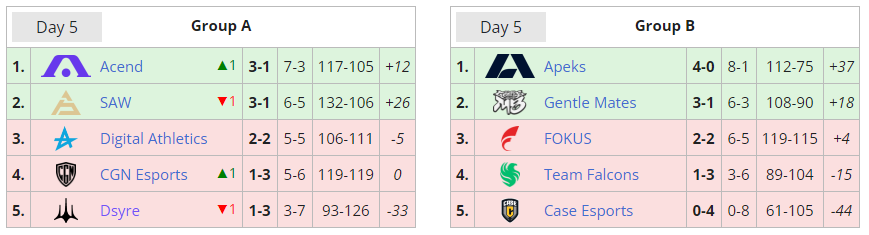This image features two distinct columns, each representing a different group: Group A and Group B. Both columns are organized under a header that reads "Day 5" in a gray box.

In Group A:
1. Position 1 is occupied by "Ken," highlighted in purple.
2. Position 2 features "Saw," marked with a yellow triangle.
3. Position 3 displays "Digital Athletics," signified by a blue star.
4. Position 4 includes "CGN," represented by a small shield, with the full name "CGNS Esports."
5. Position 5 lists "Dysere" (spelled D-S-Y-R-E) along with a small symbol.

Directly underneath these positions, there are four rows of numbers providing various statistics.

In Group B:
1. Position 1 is held by "Apex."
2. Position 2 lists "Gentlemates."
3. Position 3 includes "Focus."
4. Position 4 features "Team Falcons."
5. Position 5 shows "Case Sports."

Similar to Group A, Group B has four rows of numbers underneath these positions, offering various statistics for each team.